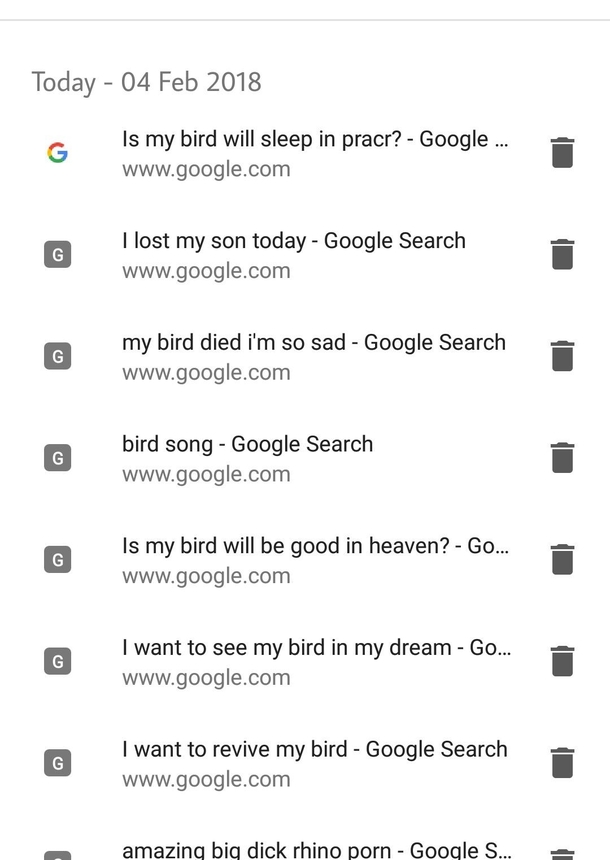In the provided image, a Google search history is displayed with a list of queries made by the user. At the top of the interface, a horizontal gray line spans across the screen. Just below this line, the date "today-04-feb-2018" is prominently shown. Following this, the image is organized into individual search entries.

The first search entry features the familiar multi-colored (red, yellow, green, and blue) Google "G" logo, representing a standard Google search. For subsequent entries, a grayed-out "G" logo is present. Each entry is accompanied by a gray trash can icon on the right-hand side, indicating the option to delete the specific search from the history.

The list of search queries includes:

1. "is my bird will sleep in PRACR" - www.google.com
2. "I lost my son today" - Google search
3. "My bird died, I'm so sad" - Google search
4. "Bird song" - Google search
5. "my bird will be good in heaven" - Google search
6. "I want to see my bird in my dream" - Google search
7. "I want to revive my bird" - Google search
8. "amazing big dick rhino porn" - Google search

Each query reflects the diverse and, at times, deeply personal nature of the user's searches, ranging from concerns about a pet bird to more unusual and explicit content.